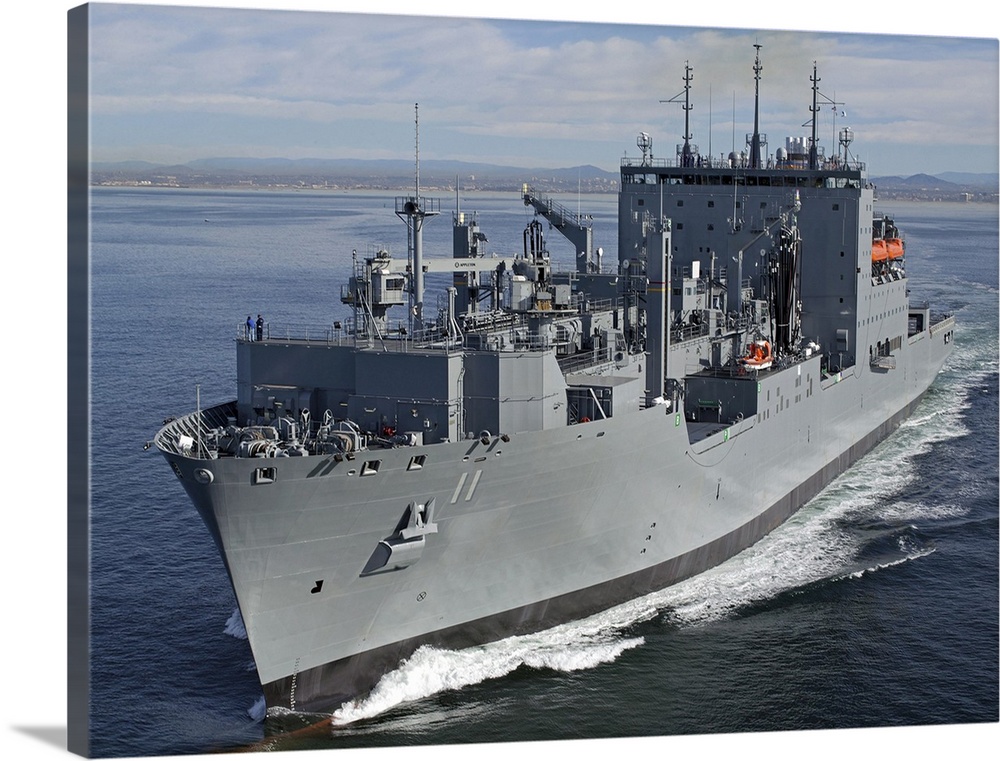This image is a photograph of an imposing, large, gray carrier ship, printed on a 3D stretch canvas frame, giving it added depth and dimension. The canvas print clearly shows the ship moving through blue waters, as evidenced by the foam and ripples along its sides. The ship features numerous metal machinery pieces, cranes, elevated surfaces, antennas, and wires, contributing to its intricate and industrial appearance. Despite its complexity, there is no indication of the ship's name or country of origin. The scene is set on a clear day with blue skies and thin white clouds. The background showcases a scenic landscape of mountains and a faintly visible shoreline, possibly including a village or city. The ship's gray color is complemented by a single black stripe at its base where it meets the water. Despite its busy structure, no people are visible on the ship.